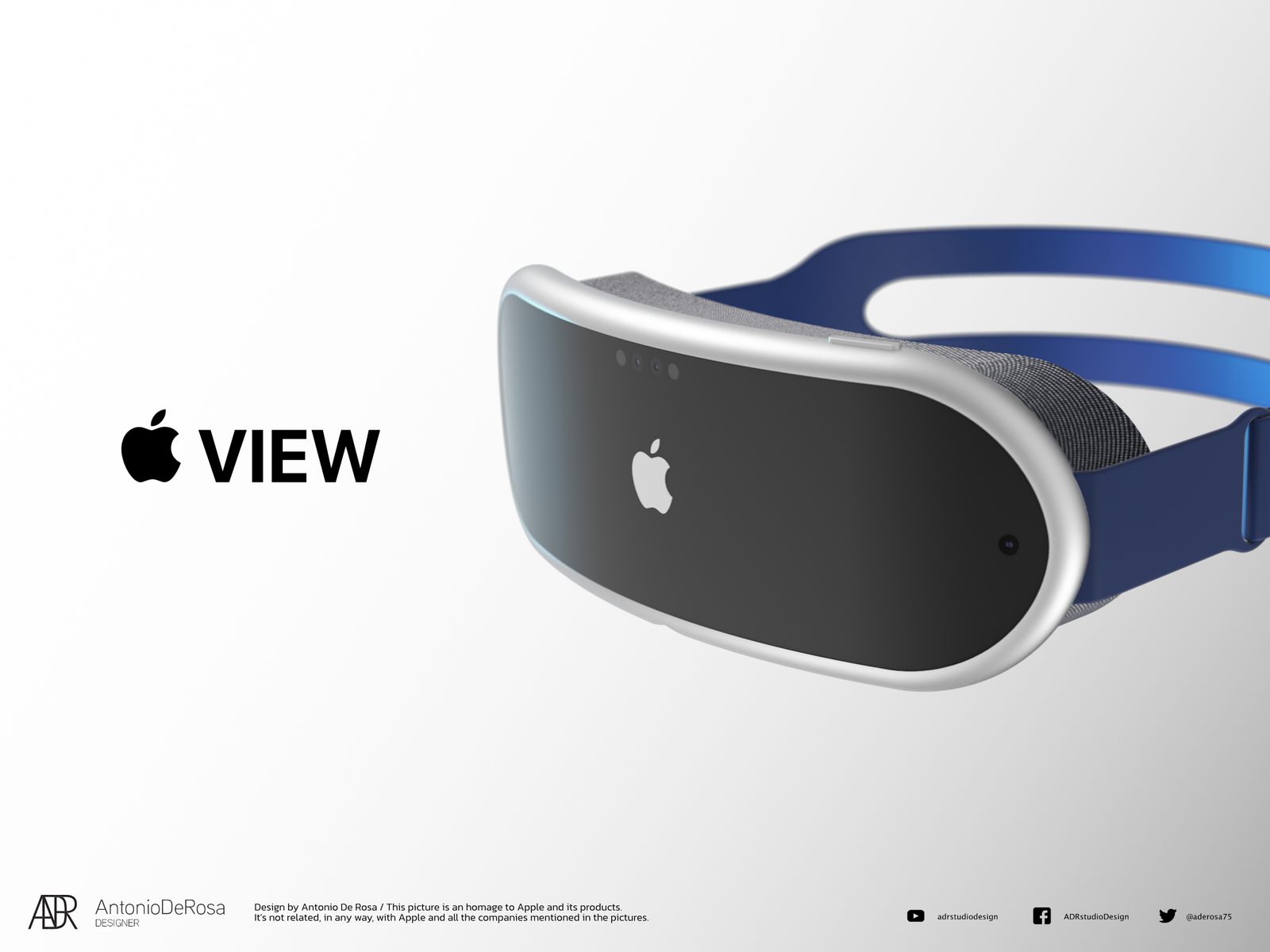The image features a detailed close-up of a concept box for an Apple-branded virtual reality headset, named "Apple View." The headset stands out with its striking design: a blue strap, gray and black cushioning, and a silver body with a black front panel. Prominent on the front is a white Apple logo, surrounded by several camera-like sensors positioned at the top and sides. The image background is blank and white. To the left of the headset, there is a black Apple logo accompanied by the word "VIEW" in black text. At the bottom right corner, there are icons for YouTube, Facebook, and Twitter, each labeled with "ADR Studio Design" and "ADEROSA75" for Twitter. This visual is the creation of designer Antonio De Rosa, serving as a homage to Apple's design language. It’s important to note that this is an artistic concept and not an official Apple product. The text at the bottom confirms it is not affiliated with Apple and that it is designed by Antonio De Rosa.